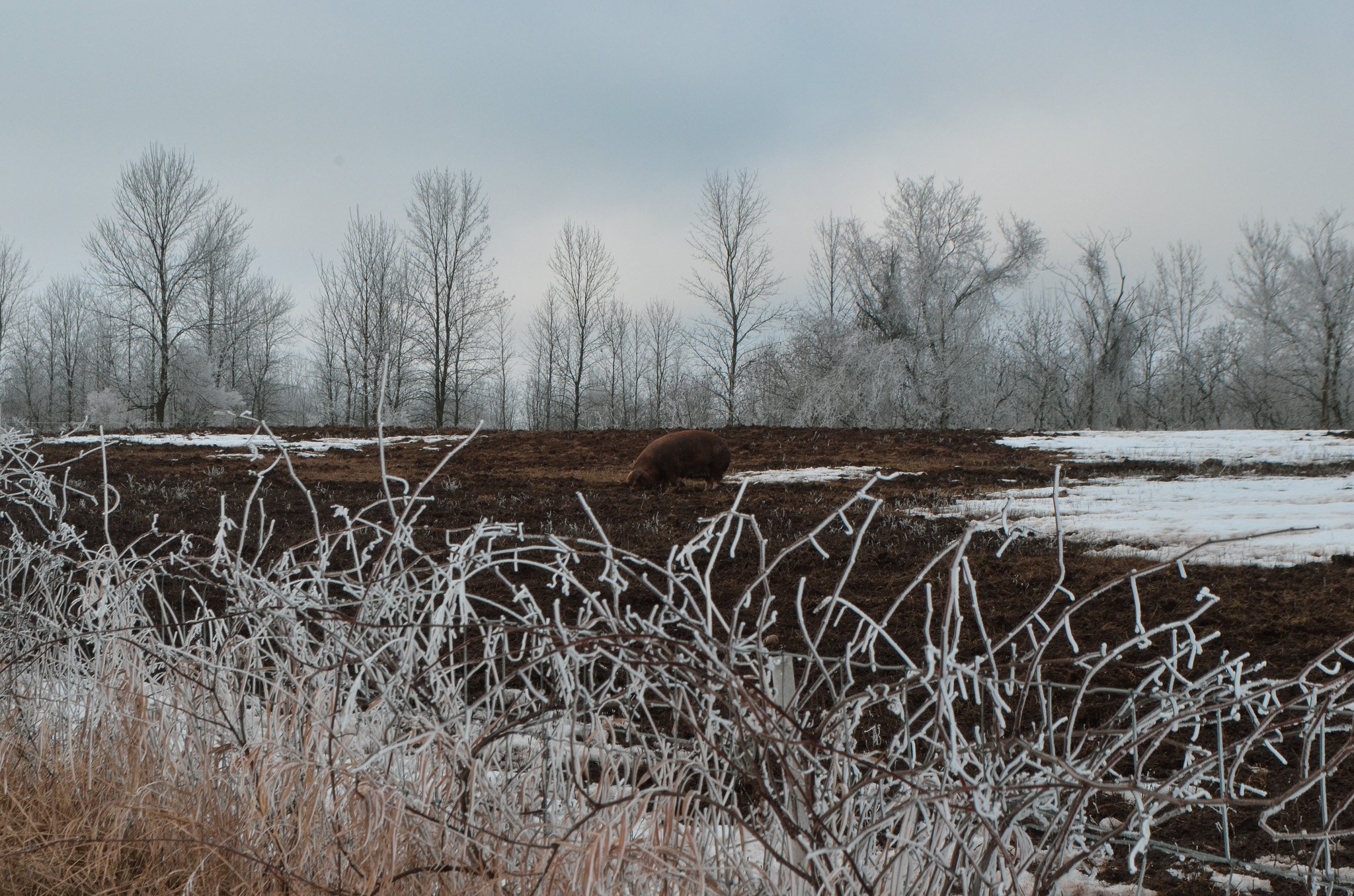The photograph captures a stark, winter scene on a very cloudy day with no visible sun. The sky is an overcast whitish-gray, contributing to the overall solemn atmosphere. In the background, a dense line of leafless, very tall trees stretches across the frame, reinforcing the wintery setting. 

In the foreground, old weeds and bushes, completely devoid of leaves, form a barrier covered with frost and ice crystals. Among this icy brush, a wire fence runs horizontally, adding to the scene's rustic charm. A log, dusted with patches of white frost, spans the width of the photograph vertically.

In the middle of the image, behind the frost-coated bushes, stands a lone animal—possibly a hog—rummaging in a large, dirt-filled field with scattered patches of snow. The animal’s brown hue blends seamlessly with the unsnowed portions of the land, further emphasizing the monochromatic and subdued palette of this wintry landscape.